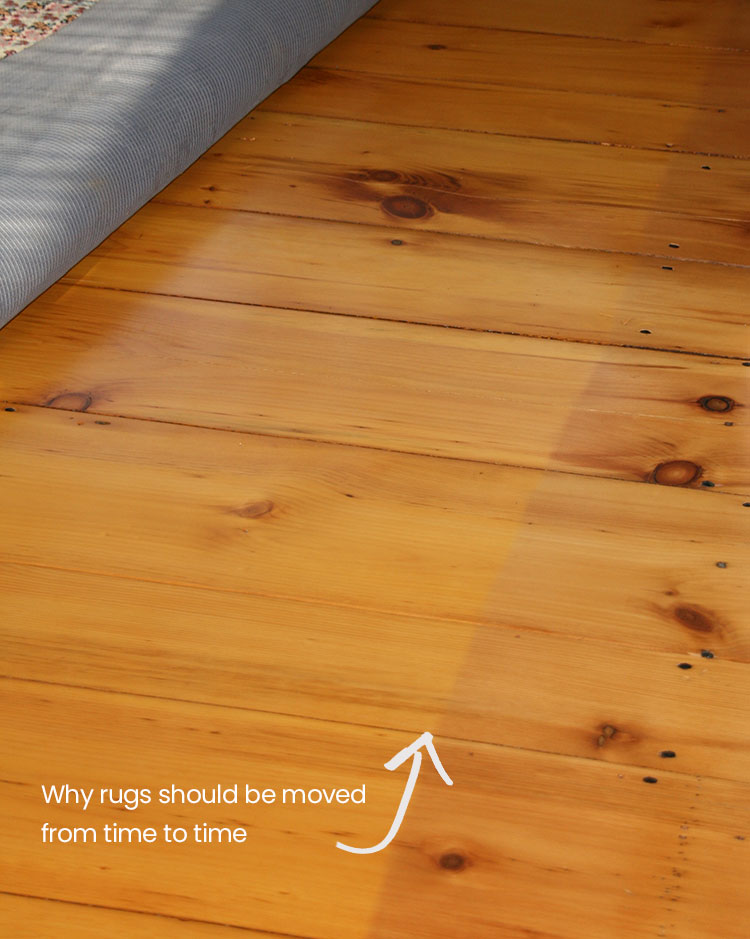This image, taken indoors, features a large section of pine wood flooring composed of planks with a light finish. Distinguishable by its light color with some staining, the flooring showcases natural knots and visible nails. In the upper left corner, a rug with a bluish backing is rolled up, revealing part of its colorful pattern. A clear demarcation exists between the lighter area under the rug and the darker, aged portion of the floor exposed to light. Near the bottom, white text accompanied by an arrow points to this contrast and reads, "why rugs should be moved from time to time," highlighting the difference in floor coloration due to prolonged rug placement.